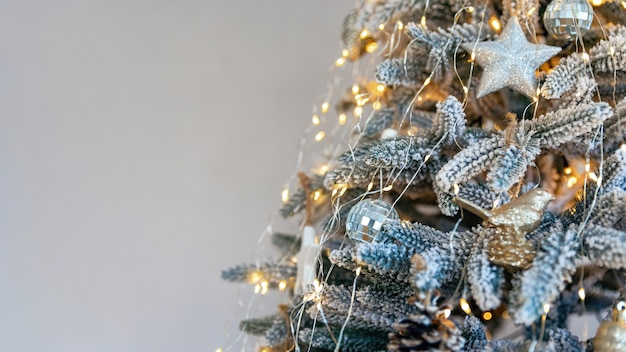The picture captures a close-up, detailed view of the right side of a flocked Christmas tree set against a fully white background. The left half of the image is blank, drawing attention to the tree adorned with various decorations. The Christmas tree, primarily white with hints of green needles, is adorned with fake snow, giving it a frosted appearance. The decorations include gold star ornaments, silver disco ball ornaments, and strands of yellow twinkle lights that add a warm glow. Tinsel drapes across the branches, enhancing the festive look, and a pine cone can be seen near the bottom right of the tree, adding a natural touch. Notably, the image features a mix of authentic-looking needles and possible plastic ones, contributing to the overall white and gold color scheme.